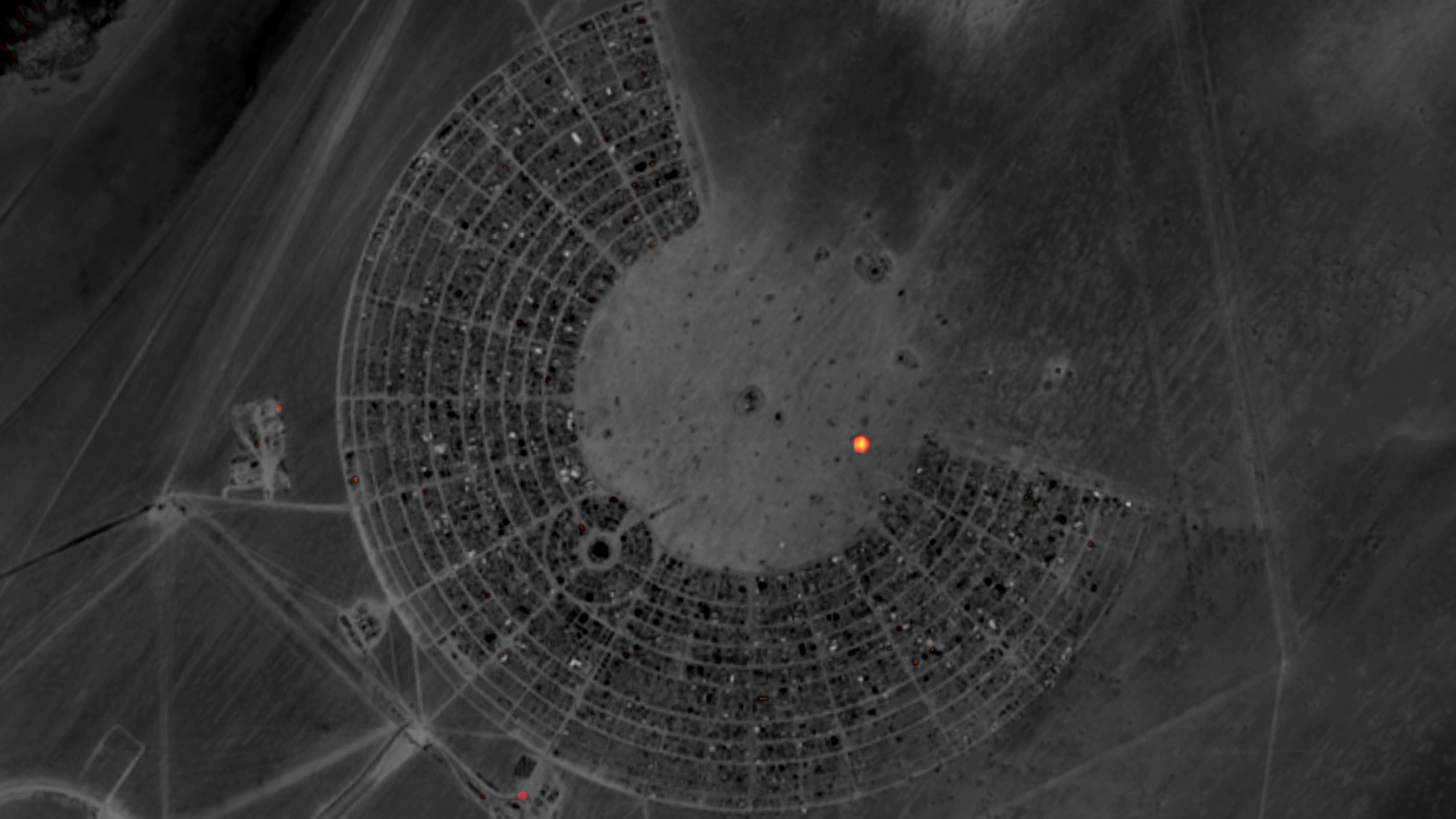The image appears to be an aerial photograph taken from above, featuring a dark outdoor setting. The focal point of this image is a large, C-shaped formation that resembles either the stands of a stadium or a set of city streets. Within the center of this C formation, there's a gray patch, highlighting a complex design composed of circles within circles, overlaid with dark gray lines and splotches. 

Prominently displayed in the middle of this formation is a bright, neon orange dot, which stands out against the predominantly gray backdrop. Additionally, there are noticeable red dots, one of which is located toward the center bottom of the image, appearing as a dark red light, and another on the left side, accompanied by two other dots that are varying shades of red and brown. Surrounding these central elements, light gray foam-like swirls extend outward, particularly towards the right side of the image, adding texture and depth. 

The bottom right corner of the photograph is noticeably darker with gray and white markings, providing a stark contrast to the lighter elements within the central patch. Overall, the image's intricate details and varying shades of gray, punctuated by the distinctive red and orange dots, create a visually compelling composition.